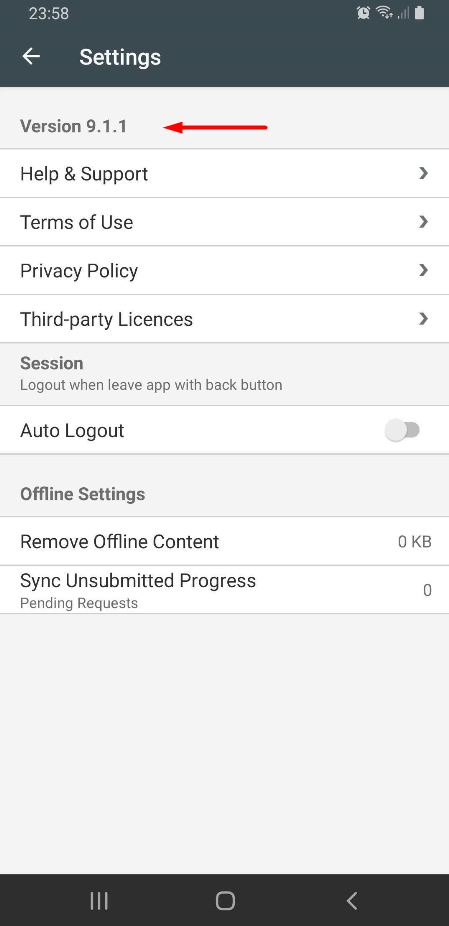In the image, there is a smartphone screen with a black border at the top displaying the time "23:58" and a single signal bar next to an alarm clock icon. Below this, a white left-facing arrow and the word "Settings" in bold white letters are prominently displayed. 

The settings menu is organized into several sections with each item separated by a light gray line. The first line reads "Version 9.1.1," marked by a red arrow pointing to the left. The subsequent lines list the following options: "Help and Support," "Terms of Use," "Privacy Policy," and "Third Party Licenses."

The next section features a gray background box labeled "Session," with a note that reads "Logout when leave app" accompanied by a back button. Below this, another section with a white background box labeled "Auto Logout" includes a toggle switch on the right, which is set to the off position (indicated by a gray color).

Further down, a gray box reads "Offline Settings," and underneath it, a white box states "Remove Offline Content (0KB)."